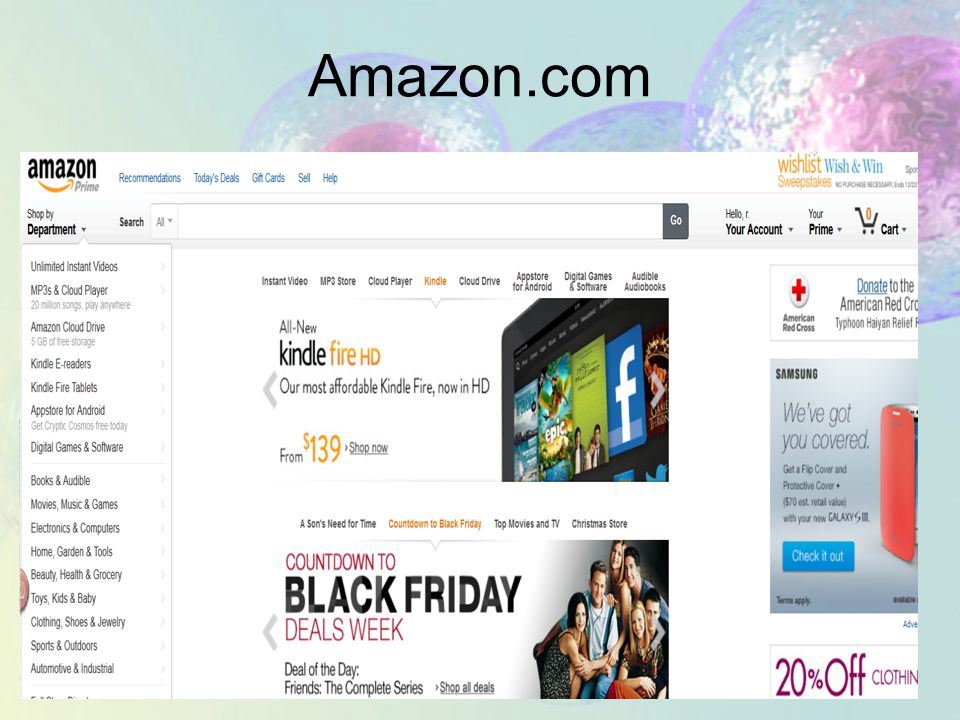This is a detailed screenshot from an old version of the Amazon.com website. The screenshot appears to be quite dated, as it does not resemble the current layout of the site. The image is cropped oddly at the top, where "amazon.com" is displayed in a simple font against a background featuring a 3D CGI graphic of what appears to be cells with nuclei. There are three large transparent spheres containing smaller purple spheres.

The visible part of the page features the Amazon Prime logo at the top left, along with website navigation tabs labeled Recommendations, Today's Deals, Gift Cards, Sell, and Help. On the top right, there are options for Wishlist, Sweepstakes, and Wish and Win. A welcoming message in the top right reads "Hello" with the user's name blurred out, followed by options for "Your Account," "Your Prime," and "Cart," which indicates that the cart is empty with a count of zero.

The main section of the screenshot highlights a few offers, notably "Kindle Fire HD, Our Most Affordable Kindle Fire Now in HD" with an image of the Kindle and a price starting from $139, along with a "Shop Now" button. Below that, there's a banner announcing "Countdown to Black Friday Deals Week" and a "Deal of the Day" featuring "Friends: The Complete Series." There is also a smaller tag encouraging users to "Shop All Deals."

On the right side, advertisements are visible including a Samsung promotion, a 20% off clothing sale, and a call to "Donate to the American Red Cross." On the left, under the Amazon logo, there's a "Shop by Department" section with a drop-down menu expanded to show various department choices, although the specific departments are not mentioned in the description.